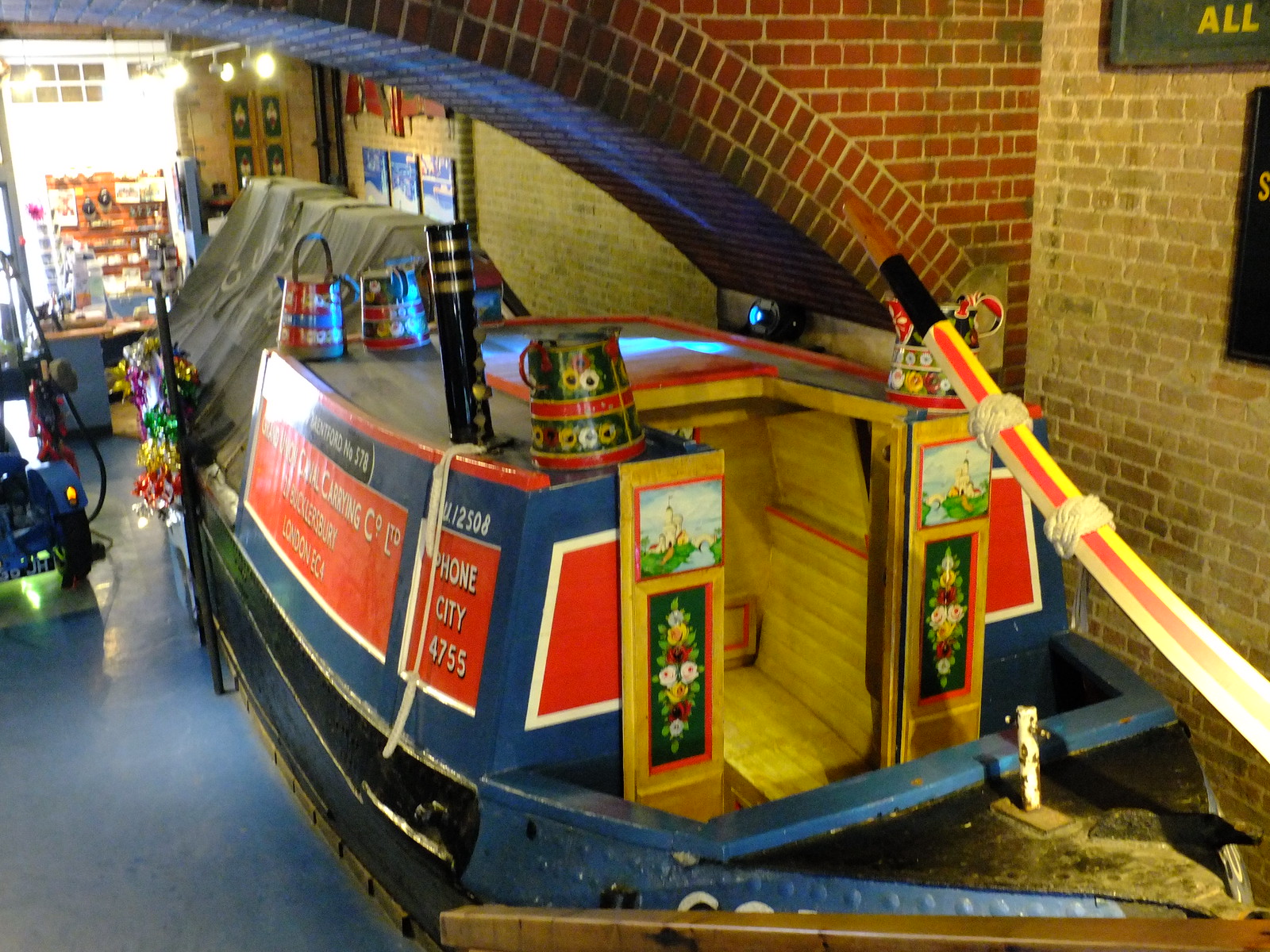Inside a large brick building that resembles a cross between a hardware store and a museum gift shop, a vibrant display captures attention. A blue canal boat with “London, Bond City” inscribed on it is the centerpiece. Adorned with red and white detailing, the boat features a yellow cabin area, equipped with a small seating space and a long handle for steering. To its right, partly obscured, stands a significant piece of equipment, hinting at the building's practical uses. The boat is situated next to a brick wall, under a large brick archway, which enhances the display's grandeur. In the distance, the cash register area is bathed in natural light from a large window, adding to the bright, sunny ambiance of the scene.